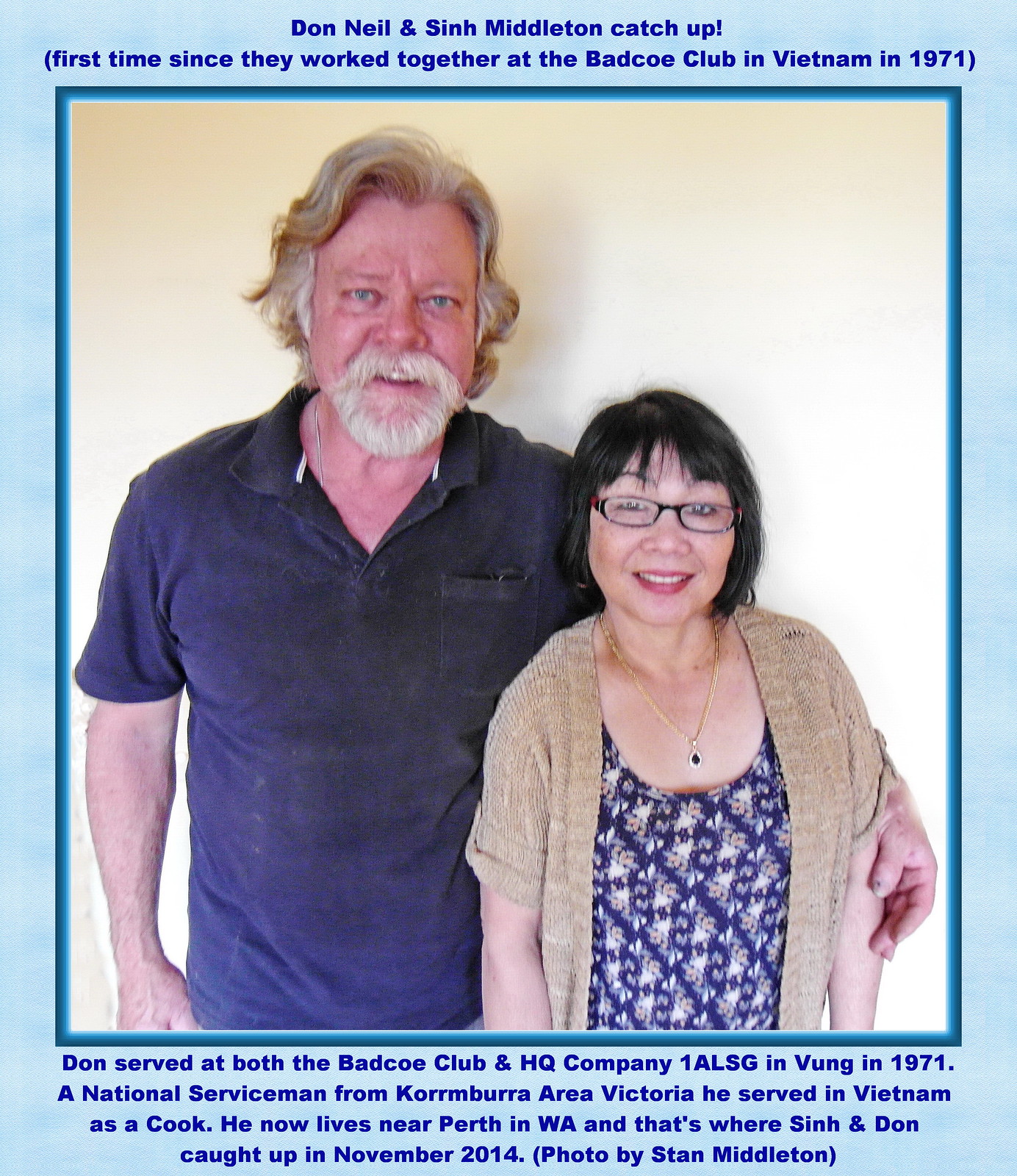The image is a color photograph featuring two people standing side by side, both facing the camera. On the left is a white male with partially gray, partially dirty blonde shaggy hair around his ears. He has a very pink complexion, blue eyes, and a white goatee. He is wearing a dark blue collared polo shirt. On his right stands an Asian female with lighter skin, short black hair styled in a bob with bangs. She wears dark-rimmed glasses and red lipstick. Her outfit consists of a blue top with white flowers, covered by a beige cardigan. The photo is bordered by a soft light blue color. Dark blue lettering at the top of the image reads, "Don Neal and Sinh Middleton catch up. First time since they worked together at the Batco Club in Vietnam in 1971." At the bottom, it states, "Don served at both the Batco Club and HQ Company 1ALSG in Vung in 1971. A national serviceman from Kurumba area, Victoria, he served in Vietnam as a cook. He now lives near Perth in WA, and that's where Sinh and Don caught up in November 2014." The photo credit is given to Stan Middleton.